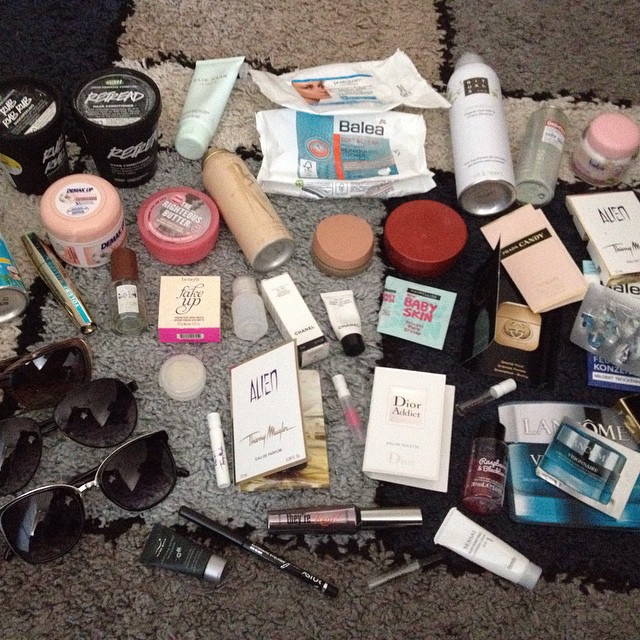A diverse assortment of beauty and skincare products is casually arranged on a carpet with shades of brown and gray, featuring both dark and light variations. The collection includes items from multiple brands such as Alien, Fake Up, Dior, Baby Skin, Balea, Retread, and Lancôme, among others that are indistinguishable due to picture quality. The products vary in type, with an emphasis on smaller items like lipsticks, tiny bottles, and eye pencils. Amidst the beauty items, three pairs of sunglasses are also scattered. The arrangement lacks any specific order, contributing to the eclectic, haphazard display on the textured carpet.